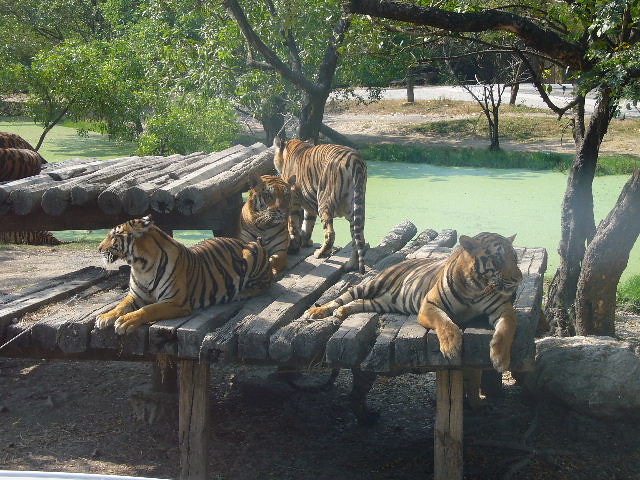The image showcases a habitat within a zoo that serves as a haven for tigers. Centered on a multi-level wooden structure, constructed with logs and elevated on sturdy stilts, the scene features four majestic tigers. Three of these tigers are lounging comfortably on the first level, with their attentive gazes directed towards the camera. The fourth tiger stands slightly apart on the higher tier, facing away towards the backdrop, which features dense trees and a body of greenish water. The setting is spacious and naturalistic, bordered by verdant foliage and trails likely used by their keepers. On a closer look, there might be additional tigers partially visible on the higher level to the far left, hinting at the presence of even more big cats enjoying this expansive, outdoor enclosure.